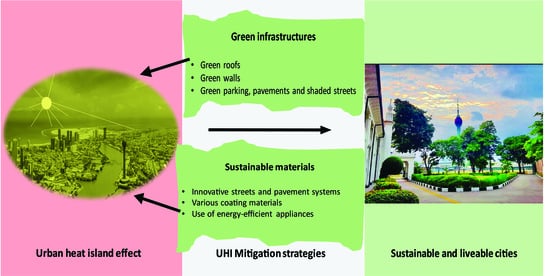The image is a comprehensive diagram divided into three sections, each interconnected to convey the importance of green infrastructure and sustainable materials in combating the urban heat island (UHI) effect. The left section features a pink background with a green oval containing an aerial view of a city with a sun overhead, labeled "Urban Heat Island Effect." The cityscape depicted here is somewhat greenish in tone. 

The middle section, set against a white background with two green stripes, lists various green infrastructures such as green roofs, green walls, green parking, and shaded streets. Below this, it mentions sustainable materials, including innovative pavements, various coating materials, and energy-efficient appliances, under the heading "UHI Mitigation Strategies."

The right section showcases a greener perspective: a city scene with a clear blue sky, vibrant green grass, and an abundance of trees, suggesting the benefits of such sustainable practices. Arrows from the middle section connect to both the left and right images, visually linking the concept of green infrastructures and sustainable materials to the goal of creating more sustainable and livable cities.